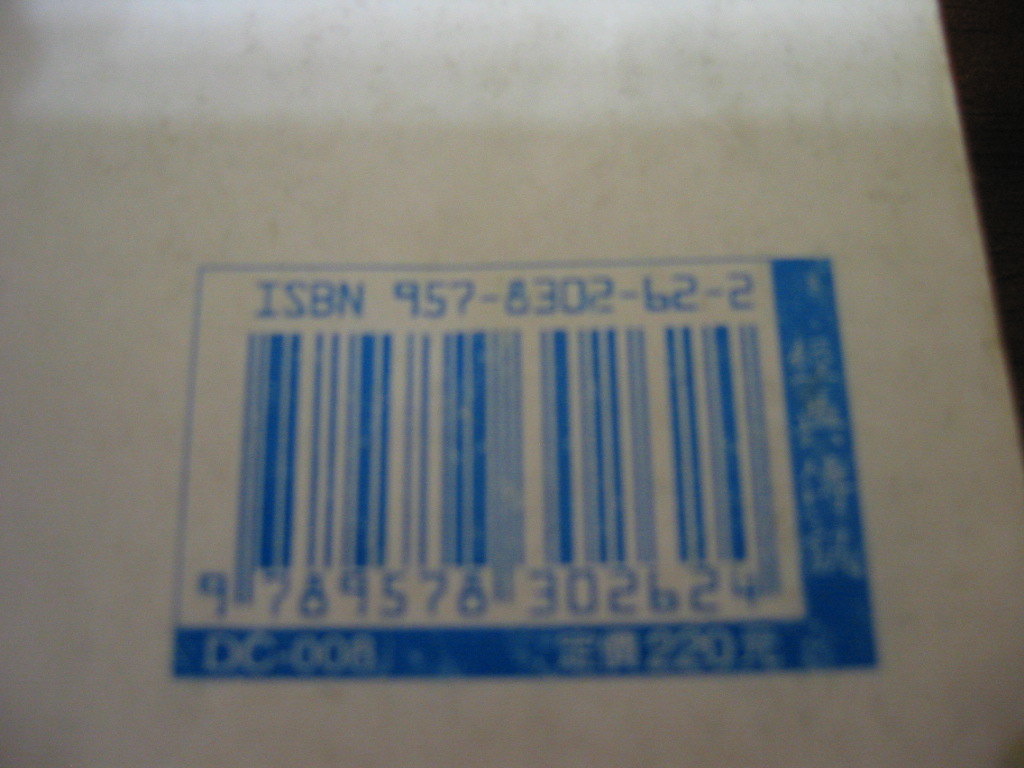This slightly out-of-focus image features a barcode situated in the bottom right corner. The background is predominantly black, providing a stark contrast to the white barcode. Above the barcode, there is blue text displaying the ISBN number "957-8302-62-2" and just below the barcode, the number "9789576302624" is visible. A thick blue border runs along the bottom and right side of the image, framing the barcode. At the bottom of the border, the letters "DC" and the number "220" are printed in blue. Additionally, there are white characters in what appears to be an Asian script positioned to the right of the barcode, adding a layer of complexity to the image’s details.